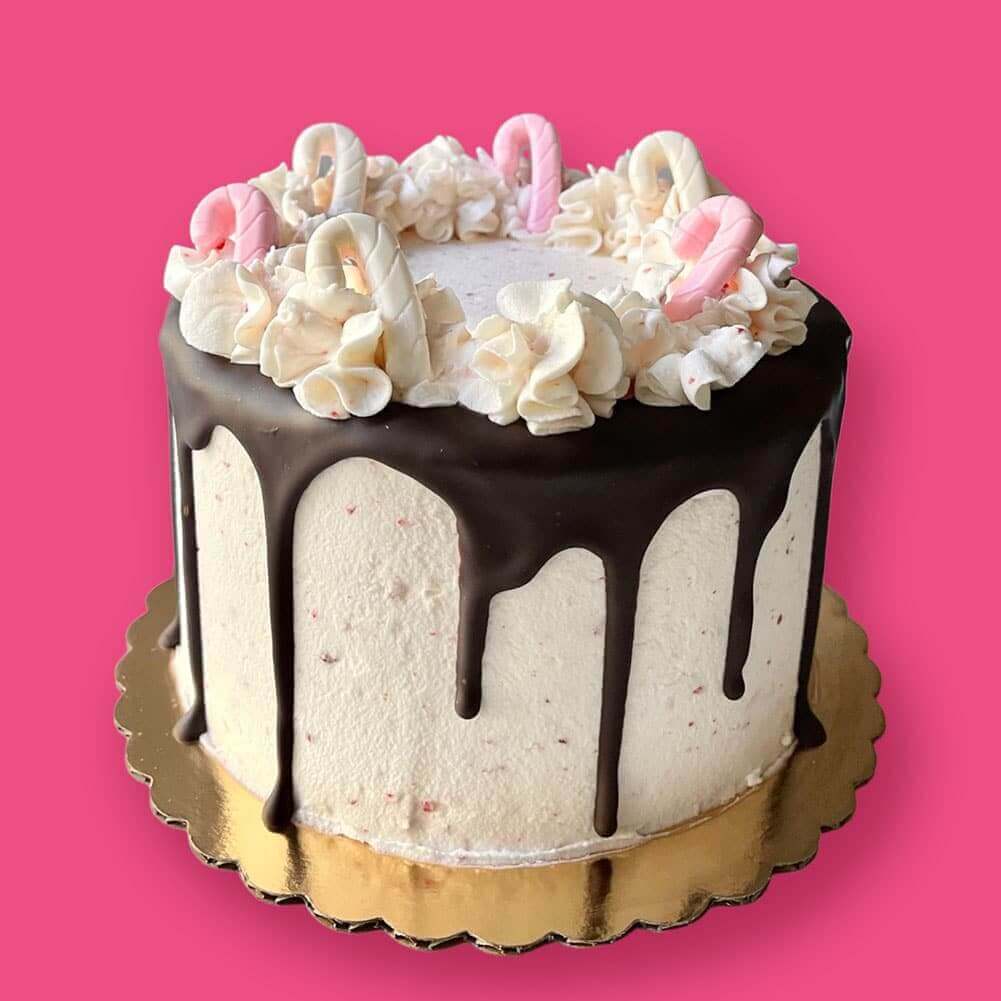This professionally taken color photograph showcases a beautifully detailed, cylindrical cake set against a bright pink background, enhanced by its gold scalloped-edged platter. The cake, appearing somewhat like the top of a top hat, features a buttercream-colored frosting with a refined aesthetic. Hardened chocolate sauce is artistically drizzled around the top, cascading down the sides in stylized drips. Atop the cake, decorative puffs of off-white frosting are neatly arranged along the edge, interspersed with candy canes. These candy canes alternate between white and a pinkish hue, bringing a festive vibe to the presentation. Additionally, the textured surface of the cake has speckles of red and brown and gives an impression of smooth ice cream, adding to its rich and enticing appearance, suggestive of peppermint flavor.